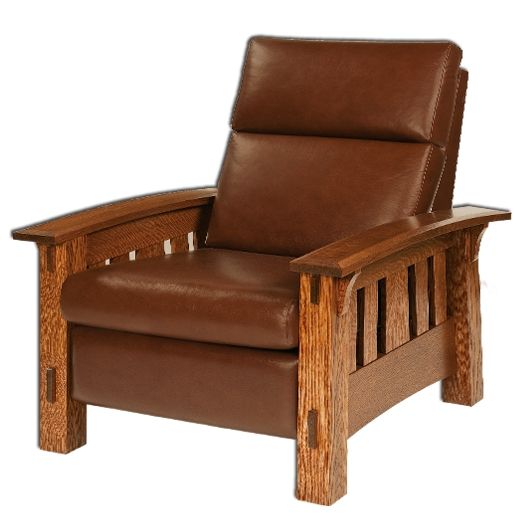The image depicts a beautifully crafted Mission-style reclining chair, blending both wood and leather elements. The chair features a robust wooden frame with light-toned 4x4 legs that contrast subtly against the darker wood of the armrests and side slats. The sides of the chair showcase vertical wooden slats that are evenly spaced, adding a touch of elegance to the design. The chair is upholstered in rich, medium-brown leather that looks soft and inviting. The headrest appears puffy, providing extra comfort, while the backrest is slightly flatter. The chair is designed with four stitched-together cushions, which enhance its plush feel. Additionally, there seems to be a mechanism to extend the footrest, indicating its capability to recline. It's a wide and accommodating chair ideal for relaxation, with flat wooden armrests for easy resting. The entire setup is staged against a white background, highlighting the chair's intricate details and polished finish.